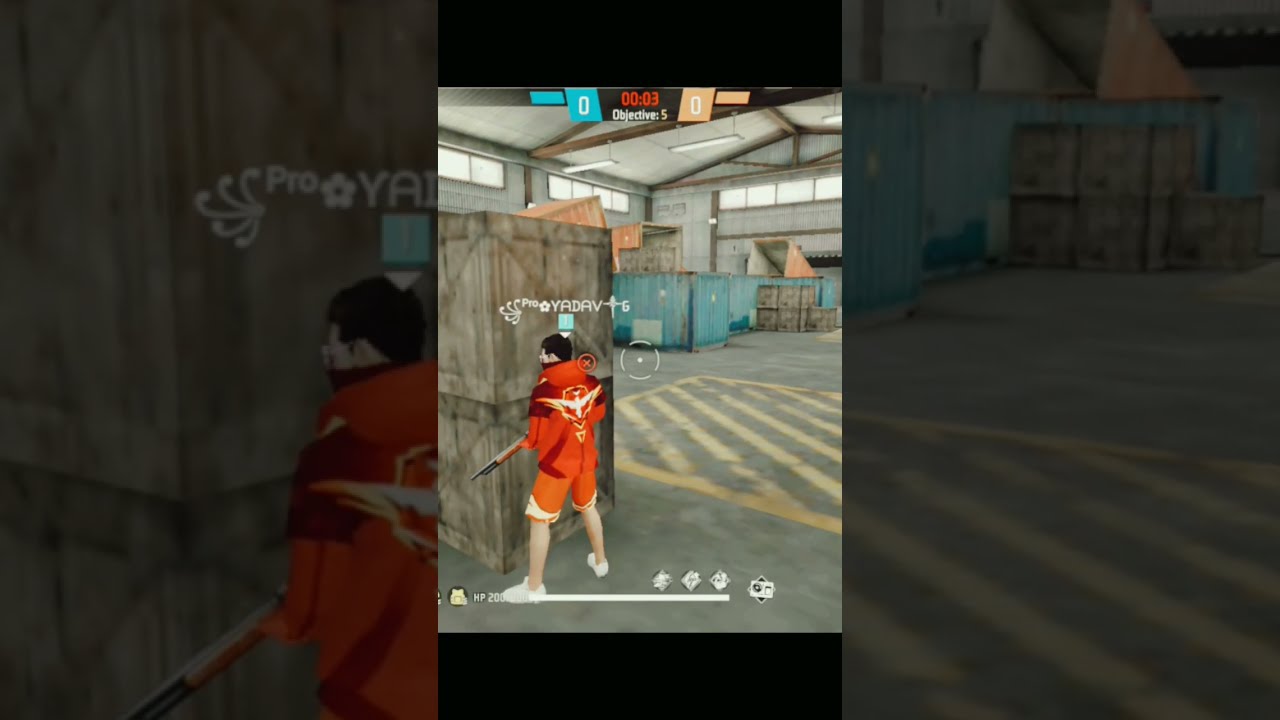The image is a detailed screenshot from a video game, set in a dimly-lit industrial environment, possibly a warehouse or parking garage, with a concrete floor featuring yellow stripes. In the center stands a man with light skin and black hair, wearing a burnt orange shirt with a white phoenix symbol on the back, and dark red shorts with gold trim. He has on white running shoes and appears to be holding a long gun or rifle. The scene includes large blue dumpsters and various stacked wooden crates and boxes. Above the man, in white font, is the name "YADAV." The image also shows a scoreboard at the top; the left side, marked in blue, displays a score of 0, and the right side, marked in orange, also shows 0. There is text indicating "00:3" and an objective "5". The background is grayed-out, with the colorful central image contrasting against an expanded version. The man’s posture and context suggest a sense of isolation and determination, hinting at a competitive scenario.